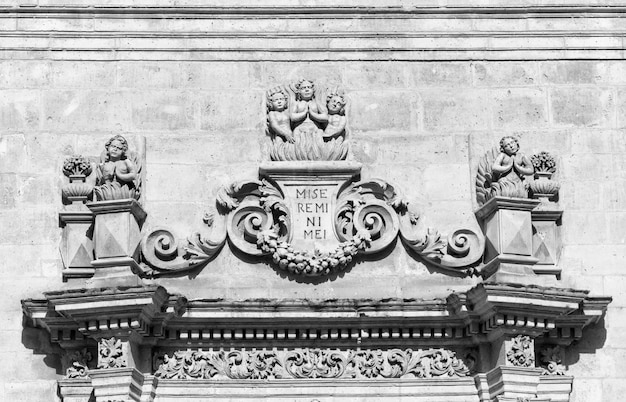The black and white photograph captures the intricate architectural relief adorning the top of a doorway on an ancient stone building, likely a few hundred years old. Constructed possibly from marble or cement, the structure features a tiered molding at the base, above which lies a richly detailed filigree decoration with ornate, leafy vine carvings. Symmetrically positioned to the left and right are box pedestals or vases, each adorned with carved children who appear to be emerging from lotus flowers. In the center of the relief, three additional child-like angelic figures, also emerging from flowers, add to the elaborate design. Above these figures, inscribed in the stone is the Latin phrase "MISEREMINI MEI," likely translating to "Have mercy on me." The overall composition suggests a sophisticated, symmetrical ornamentation typical of classical architecture, possibly indicative of a significant or governmental building.